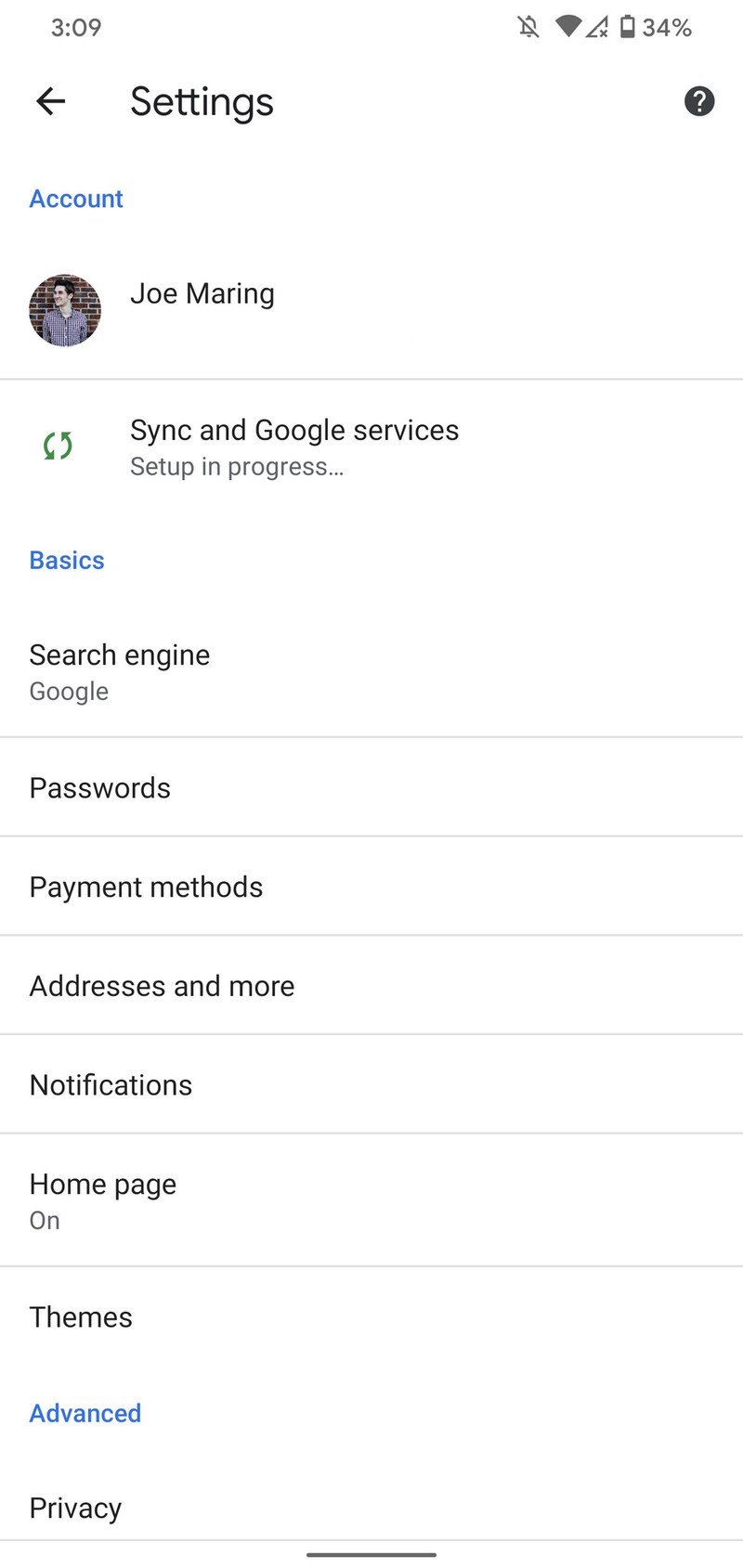The image displays the settings page of what appears to be a Google service on Joe Mehring's phone. The time displayed on the device is 3:09 PM, and the battery level is at 34%. Joe Mehring's profile information is visible, including a headshot where he is posing against a brick wall while wearing a button-up shirt. The settings page indicates that a synchronization process for Google services is currently in progress.